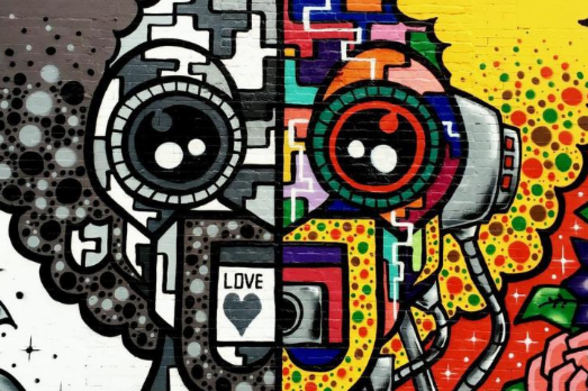The image showcases a piece of street art on a brick wall, divided vertically into two distinct halves. The left side of the mural is in black and white, depicting a large eye and a section that reads "LOVE" with a heart. Below this, there is a partial camera. The right side bursts into a vivid array of colors including green, pink, blue, yellow, and red. The artwork appears to represent a robot-like face split down the middle, with the right side also featuring a red-eye lined with green, suggesting some form of technology or android aesthetic. This colorful side is embellished with an afro-style pattern with polka dots, and a pink rose with green leaves is visible at the bottom right corner. The overall impression is that of a surreal, abstract face, blending elements of technology and street art, marked by intricate details that play with symmetry and color contrasts.